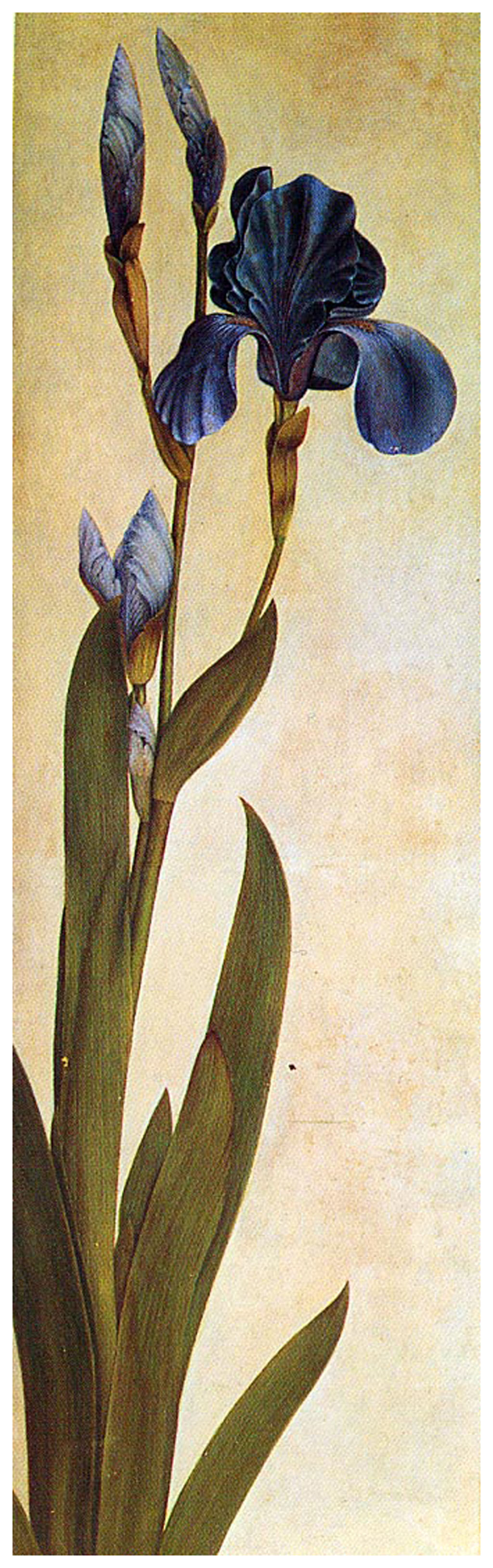This highly vertical, hand-colored drawing or painting features an elegant depiction of an iris flower. The composition is notably taller than it is wide, and the background gracefully transitions from a washed-out beige to subtle blue-gray tints. Dominating the scene is a single, central flower stalk adorned with tapered olive green leaves that rise vertically. At the apex of the image blooms a fully opened iris, its deep blue petals highlighted with touches of white. Flanking this blossom are four additional buds; one is barely beginning to open on the left, while the other three, including two at the top, remain tightly closed. The vivid green of the foliage and the intricate detailing of the petals create a striking contrast against the muted background, bringing a lively yet refined touch to the artwork.